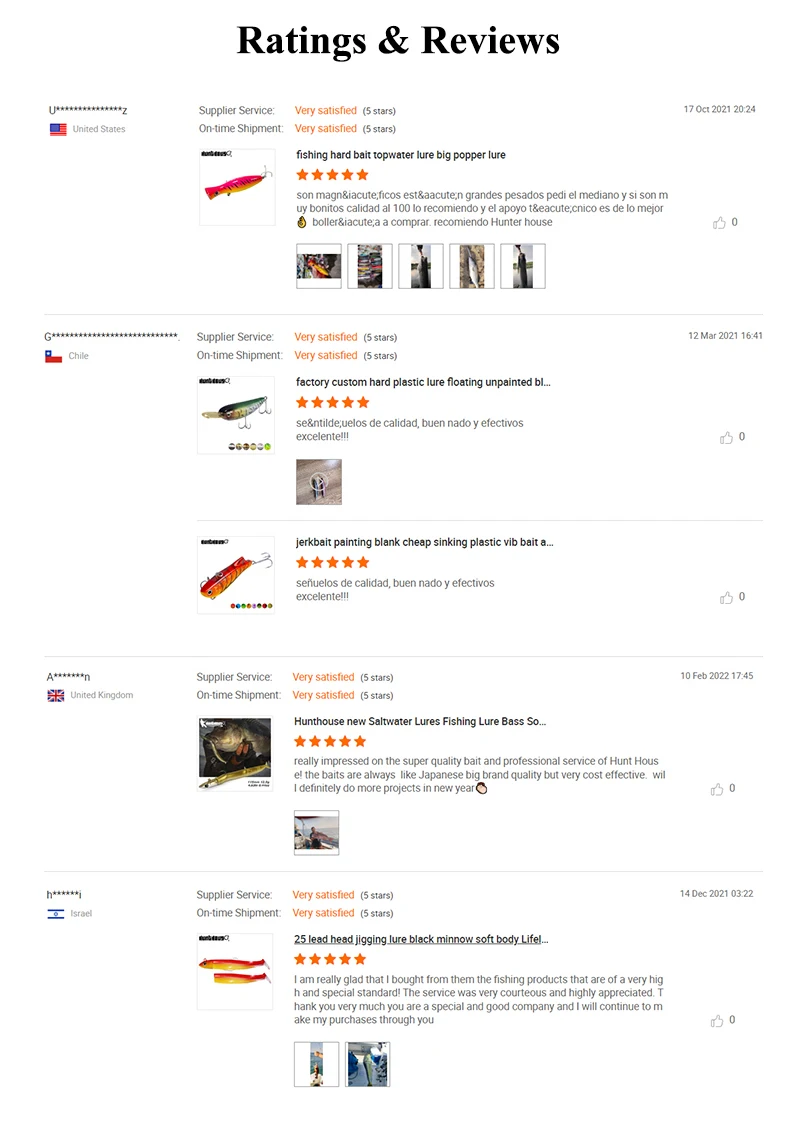The image displays an Amazon web page, focusing primarily on the "Ratings and Reviews" section, emphasized in bold. On the left side, there is a detailed review contributed by a user from the USA, indicated by the American flag icon. This user is extremely satisfied with their purchase, as reflected by their five-star ratings for both the product and the timely shipment. The product reviewed is an orange and yellow fishing lure, and the review text is highlighted in orange font. The user has also shared several pictures of the product and provided their comments in Spanish.

Additionally, there is a review from a customer in Chile, who also gives five-star ratings for both the product and the on-time shipment. This reviewer has purchased two fishing lures: one in green, yellow, and gray, and another in orange and yellow. Similar to the USA review, the comments are written in Spanish.

Another review is visible from a user in the UK, who has purchased a green and yellow fishing lure. However, further details about their review, such as star ratings and comments, are not provided in the image.